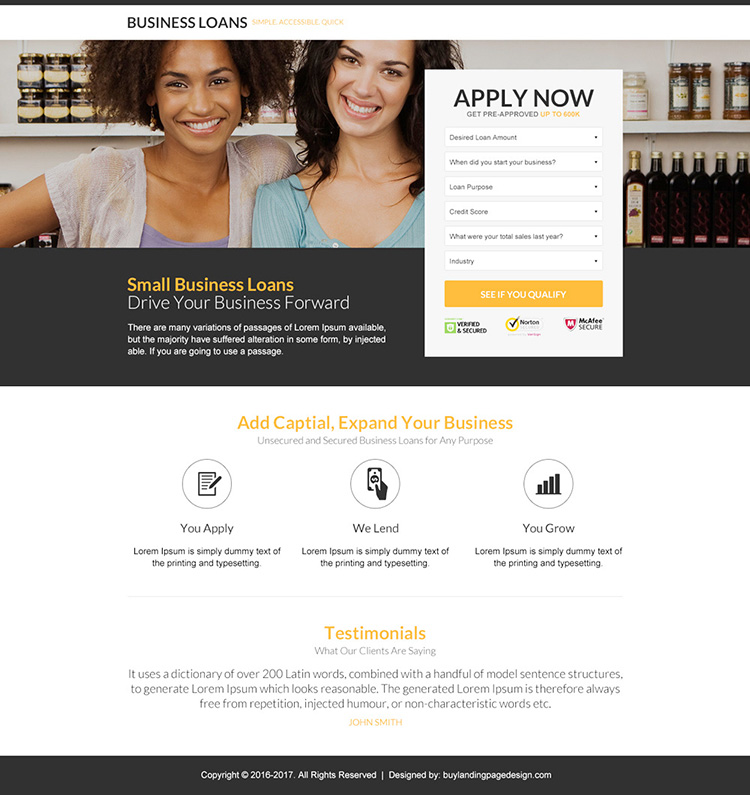The image showcases a mobile application or website page for business loans displayed on a smartphone. The header prominently reads “Business Loans” in black text, followed by the tagline, “Simple, Accessible, Quick” in yellow. Below this, a photograph features two smiling women embracing each other—one is African American with short, curly brown hair, while the other is Caucasian with dark brown, almost black hair. 

As you scroll down the page, there is a section labeled “Apply Now,” highlighted with a white rectangular input area for user information. At the bottom, a yellow rectangular button prompts users to “See if you qualify.” Additional sections include messages like “Small Business Loans: Drive Your Business Forward,” advocating for loan benefits such as adding capital and expanding one's business. The application process is simplified into three steps: “You Apply, We Lend, You Grow.” The layout also features a section for testimonials, marked in yellow, offering social proof of the service's effectiveness.